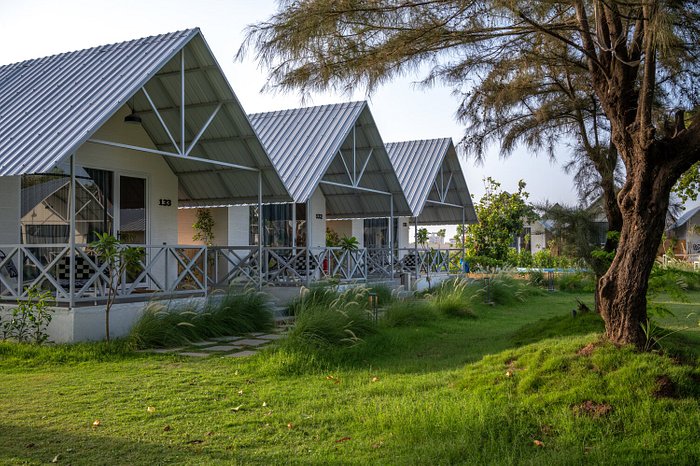This photograph captures an outdoor scene featuring three identical white buildings that appear to be either retirement or vacation homes. Each building has a distinct gray metal roof shaped like an upside-down V, and features a small white concrete porch with gray metal railings adorned with a rectangular pattern and an X in the center. The buildings are lined up next to each other, with house numbers visible but not legible.

In the foreground, there's a vibrant, well-maintained green lawn with a stone walkway bordered by tall ornamental grasses. On the far right side of the image, a large tree with brown needles, possibly indicating it is out of season or unhealthy, can be seen. The background reveals additional buildings and trees that echo the architectural style of the foreground structures. The sky is clear and blue, suggesting a sunny day, but the angle of the sunlight and the lengthening shadows indicate that it is likely early evening, around 6 or 7 o'clock.